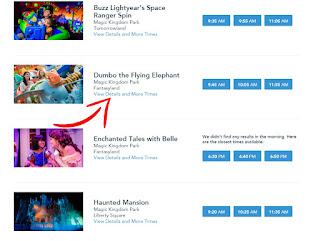### Detailed Caption:

The image appears to be a cropped screenshot of a web page, likely from a theme park's ticket or reservations section. The layout is minimalistic with four main rows, each representing a different attraction. The text and icons are quite small, making it somewhat difficult to read.

1. **First Row**:
   - **Icon**: A small cartoon image, possibly a screenshot from the ride or attraction.
   - **Attraction**: Buzz Lightyear's Space Ranger Spin.
   - **Location**: Magic Kingdom Park.
   - **Additional Information**: Below the attraction name, there's text that is not fully legible.
   - **Interactive Elements**: Links labeled "View Details" and "More Times."
   - **Available Times**: 9:35 AM, 9:55 AM, and 11:05 AM.

2. **Second Row**:
   - **Attraction**: Dumbo the Flying Elephant.
   - **Available Times**: Specific times listed similarly to the first row.
   - **Highlight**: There is a red arrow pointing to this attraction, indicating it might be of particular interest.

3. **Third Row**:
   - **Attraction**: Enchanted Tales with Belle.

4. **Fourth Row**:
   - **Attraction**: The Haunted Mansion.

Overall, this screenshot seems to be part of a booking or scheduling interface for various attractions at Magic Kingdom Park, with specific time slots available for each ride.